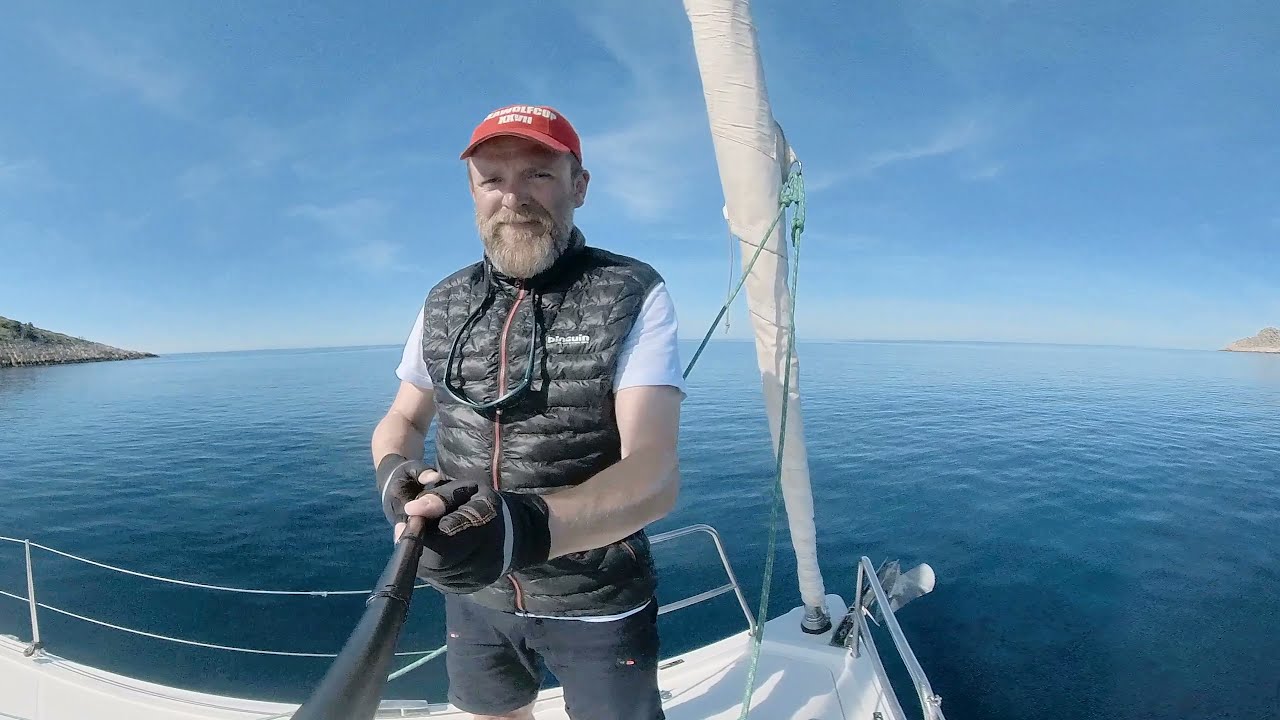In this rectangular photograph, a middle-aged man stands at the front of a white sailboat, partially holding onto metal poles jutting out from the bottom. The boat, equipped with silver railings, is set against a backdrop of an expansive body of water that transitions from light blue near the boat to deep blue further away. The water appears calm, with subtle ripples and extends to the horizon where it meets a bright blue sky, accented by wispy white clouds.

The man, likely in his 50s, has a full light-colored brown beard with a hint of salt and pepper. He wears a red baseball cap adorned with white font, a black down vest bearing a partially readable logo that resembles "Binsuin," over a white t-shirt. Around his neck hangs a pair of sunglasses. He complements his outfit with black fingerless gloves and dark, almost knee-length shorts. With a slight smile and squinting eyes, he faces the camera with a cheerful demeanor, gripping onto a black metal or tubing structure likely connected to the sailboat's apparatus. The land can be seen faintly in the upper left and right corners of the image, indicating proximity to a harbor.